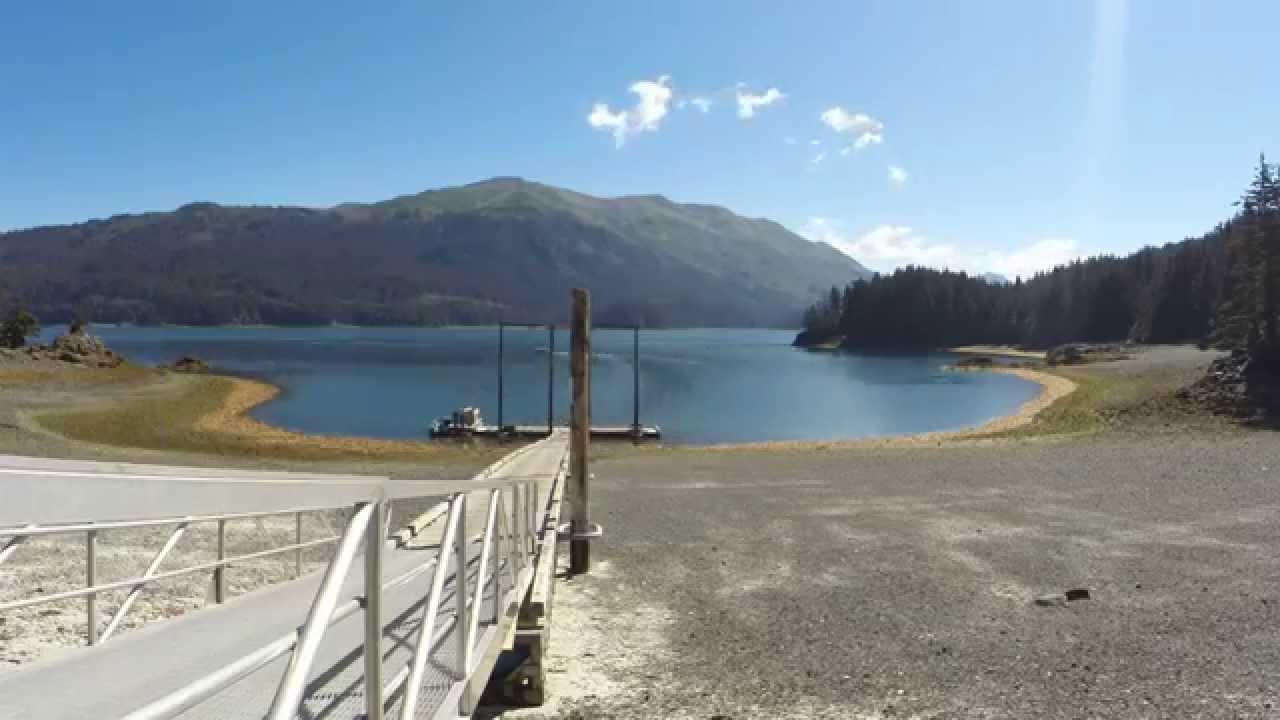In this serene image, the focus is on a tranquil, azure lake that mirrors the brilliance of the clear, sunny sky above. A long dock, adorned with white railings, extends gracefully into the still waters, inviting a leisurely stroll or reflective pause. Evidence of receded water levels is visible, where the gravel shore draws a line marking the usual boat docking point. Beyond the placid lake, a majestic mountain rises, its base cloaked in a dense forest of trees that stretch to the right of the frame. The day is beautifully sunlit, punctuated by a scattering of fluffy white clouds against the expansive blue sky, enhancing the picturesque and peaceful atmosphere.